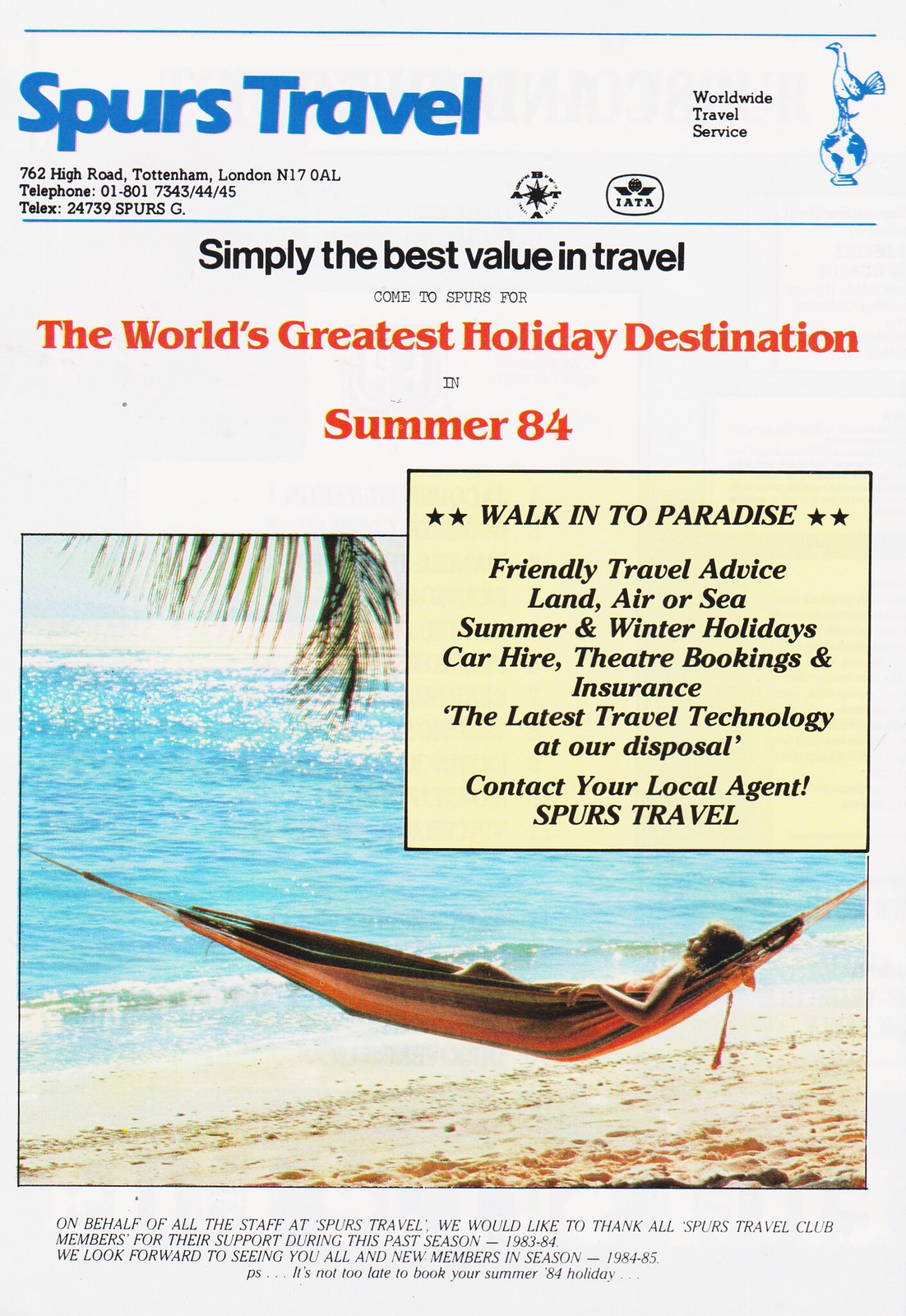This vivid travel flyer from Spurs Travel, an established agency located at 762 High Road, Tottenham, London, boasts a high-profile advertisement featuring a woman lounging in a hammock on a serene, sandy beach with crystal-clear blue water and a palm tree frond peeking from the upper left corner. The top of the off-white flyer prominently displays "Spurs Travel, Worldwide Travel Service" in striking blue letters, followed by their address, contact number, and telex in black text. The slogan "Simply the Best Value in Travel" lies just beneath. Another bold statement in reddish-orange declares, "The World's Greatest Holiday Destination, Summer 84." To the right of the relaxing scene is a detailed box that reads "Walk into Paradise," "Friendly Travel Advice," and lists various services including travel by land, sea, or air, both summer and winter holidays, car hire, theater bookings, and insurance, all backed by the latest travel technology. The footer encourages readers to "Contact Your Local Travel Agent," ensuring potential travelers know Spurs Travel is a comprehensive, reliable choice for their holiday needs.